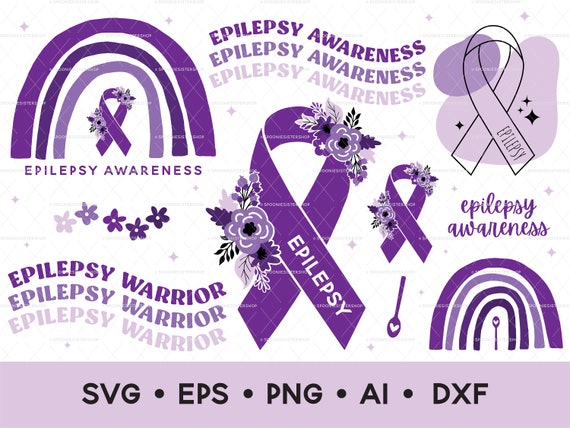This poster for epilepsy awareness is predominantly designed in shades of white and purple, with an assortment of purple-themed clip art on a white background that constitutes most of the frame. The bottom edge features a pale purple border with black uppercase text listing file formats: "SVG, EPS, PNG, AI, DXF". Above this border, the poster showcases various images and text related to epilepsy awareness. Central to the composition is a series of purple rainbow arches with a folded purple ribbon and the words "Epilepsy Awareness" below. Additional imagery includes wavy lines and several fonts spelling out "Epilepsy Awareness" and "Epilepsy Warrior", as well as other designs integrating the purple ribbon symbol. These elements collectively resemble tattoo flash art, presenting a unified collection of designs promoting epilepsy awareness.